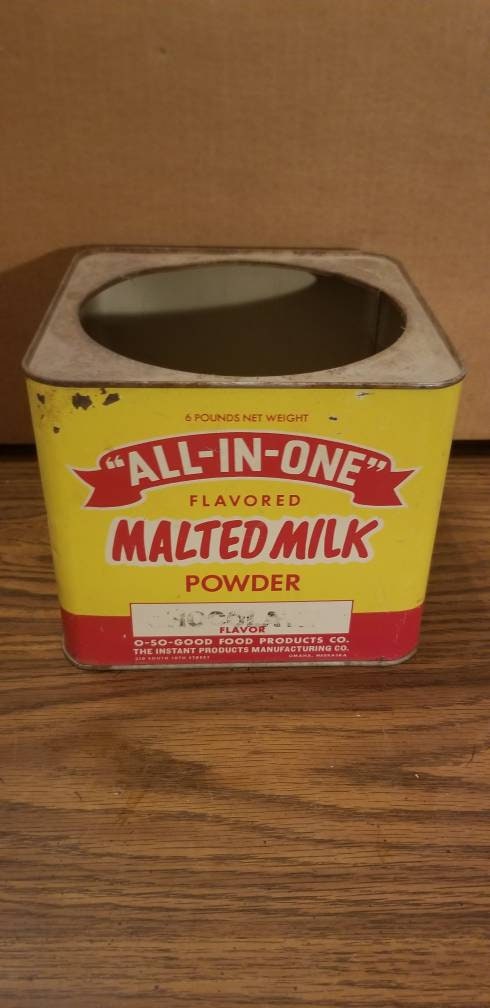This photograph features a vintage, square-shaped tin container, which once held malted milk powder. It sits on a wooden table with a cardboard box in the background, emphasizing the aged nature of the setting. The tin lacks a lid, exposing its round opening at the top. The top part of the container is a light brownish-gray, while its front is primarily yellow with accents of red at the bottom. 

The tin displays several inscriptions in a variety of colors: a prominent red banner with white letters reads "all-in-one," followed by red lettering stating "flavored malted milk powder." Below this, within a red-outlined white rectangle, some faded black writing identifies the flavor, possibly chocolate. Additional branding includes "oh so good food products CO." and "the instant product manufacturing CO." The tin's overall design, typography, and color scheme suggest it dates back 20-30 years, reflecting a nostalgic charm.